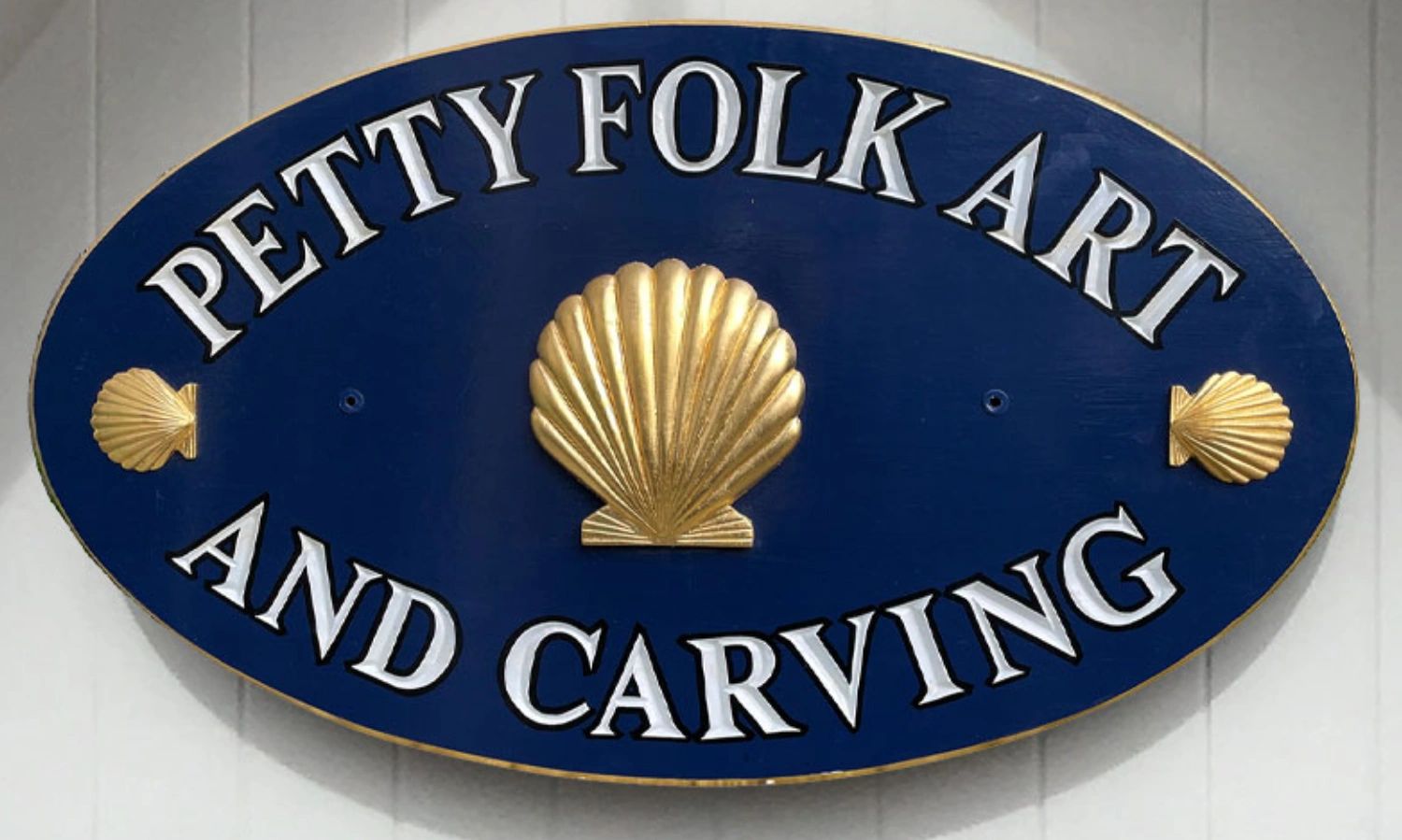The image depicts a beautifully detailed oval sign mounted on a white shiplap wall. The sign, adorned with a gold border, prominently features the text "Petty Folk Art" in a semi-circular shape at the top and "Carving" in a matching curve at the bottom. Both lines of text are engraved and painted white against a striking blue background. Three intricately designed gold seashells highlight the sign—the largest one is centered and faces upward, flanked by two smaller seashells positioned to the left and right, each facing outward. The sign appears to be metallic and casts a shadow on the white wooden panel background, indicating a light source from above. Adding to its charm, there are two holes on the sign, situated between the seashells.